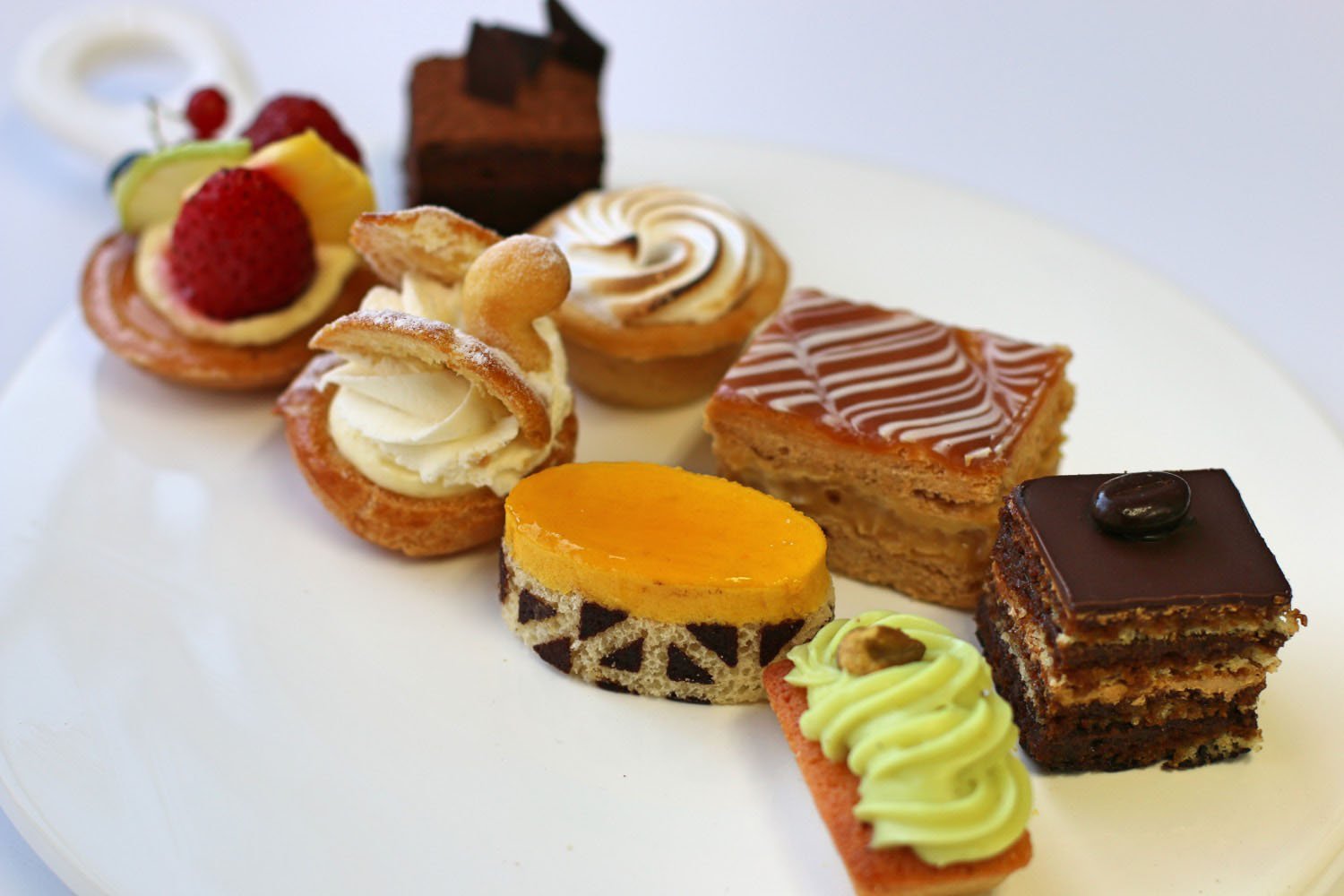Captured in natural light, the image features a white glossy plate adorned with a diverse selection of eight mouth-watering pastries. Each pastry showcases a unique and intricate design, offering a visual feast for dessert enthusiasts. From left to right, we see:

1. A rich, dense brownie, perfect for chocolate lovers.
2. A muffin with a beautifully swirled, slightly charred top, hinting at a soft and moist interior.
3. A luxurious brown cake topped with a caramel glaze and meticulously drizzled with white stripes.
4. A decadent chocolate cake crowned with chocolate-covered nuts, promising a delightful crunch.
5. A delicate pastry garnished with an assortment of colorful fruits, including a juicy strawberry and a slice of lime, adding a tangy zest.
6. A cream-filled pastry, oozing with silky sweetness.
7. A unique triangular pastry with a black and white checkered pattern, topped with velvety cream.
8. A traditional cake decorated with green piped icing and accented with a single, perfectly-placed pistachio nut.

These delectable confections are arranged on the elegant plate, which features a convenient handle at one end. The natural lighting enhances the textures and colors of the pastries, making them appear even more irresistible.